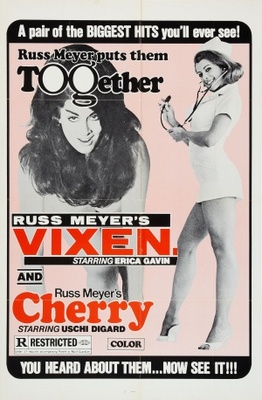This retro black and white movie poster with a light pink background features an advertisement for two Russ Meyer films: "Vixen" starring Erica Gavin and "Cherry" starring Ushi Digard. The poster has a black rectangular banner at the top with slightly curved corners that reads in bold white text, "A pair of the biggest hits you'll ever see." Below this, the central text proclaims, "Russ Meyer puts them together," with stylized "O" and "G" resembling glasses. The background appears weathered, similar to folded newspaper print with noticeable crease lines down the center.

On the right side of the image, a woman wearing an extremely short, sexy nurse's costume poses provocatively. Her white mini-dress accentuates her curves, and she has a stethoscope around her neck. To the left, another woman with a 1960s beehive hairstyle is partially visible, her body partly obscured by the text overlay. The bottom part of the poster features the films' titles in striking red text: "Russ Meyer's Vixen" and "Russ Meyer's Cherry," and it displays a restricted logo. At the very bottom, the tagline "You heard about them, now see it" emphasizes the allure of the films.